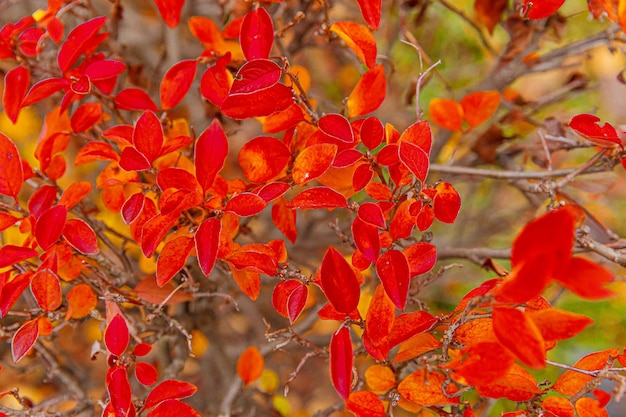The image vividly captures the essence of autumn with a dense, striking display of bright red-orange leaves, possibly from a type of shrub or small tree, occupying the entire foreground. The leaves vary in size and are attached to thin brown stems, creating a vibrant tapestry of color. The intense reds dominate the scene, suggesting the transitional phase of foliage as it prepares for fall. Scattered hints of yellow and green leaves in the blurred background add depth and contrast to the predominant red hues. The upper right corner reveals more green, hinting at unturned foliage. Additionally, a few older brown flowers can be seen on the left, merging with patches of green in the middle, further enriching the autumnal ambiance. The focused composition on the red leaves, with glimpses of the stems and blurred green areas behind, underscores the season's bright and vivid transformation.